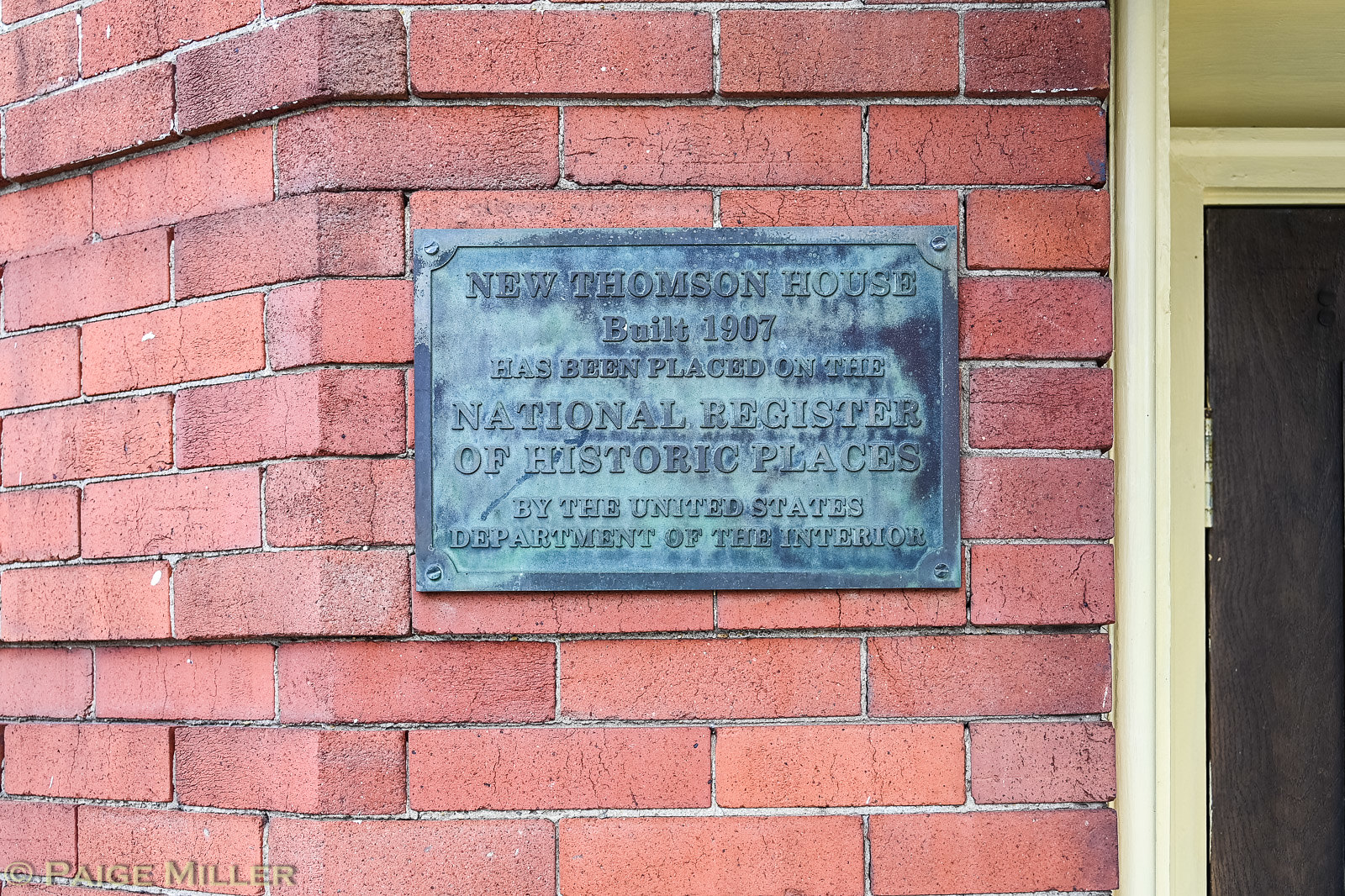This detailed photograph captures a metal plaque affixed to the exterior of a historic brick building. The background is predominantly composed of red bricks, particularly concentrated on the left and middle portions of the image. Central to the frame is a worn grayish-black plaque, significantly discolored with white spots and aging into a greenish hue over time. The inscription on the plaque, rendered in raised metal letters, reads: "New Thompson House, built 1907, has been placed on the National Register of Historic Places by the United States Department of the Interior." In the lower left-hand corner of the plaque, a copyright symbol followed by "PAIGE MILLER" is clearly visible in gray text. To the far right of the image, beyond where the brick wall ends, part of a different wall is discernible. This wall transitions from a tan color at the top to framing a dark brown door with a white painted border.